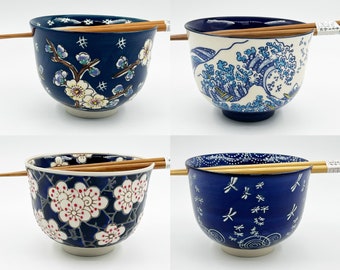The composite image portrays four distinct bowls with accompanying wooden chopsticks, arranged in a grid of four rectangular photos forming a larger rectangle. Each bowl, notable for its Japanese aesthetic and design, has a unique pattern and color palette. The bowls are designed to hold chopsticks through a specialized hole and notch, with the pointed ends resting on the edge of each bowl and oriented to the left.

In the top left, a dark blue bowl showcases a charming pattern of lighter blue and white flowers, accentuated with subtle additional marks. Adjacent in the top right, a bowl of similar dimensions features a majestic, traditional Japanese ocean wave pattern on its white exterior, with a blue interior. 

Shifting to the bottom left, the bowl displays a predominantly navy blue or black exterior adorned with delicate white and red sakura flower designs. Finally, the bottom right highlights a vibrant blue bowl encircled by an elegant white dragonfly motif.

Each bowl sits on a circular base, with distinct floral patterns and intricate designs standing out, encapsulating a balance of both traditional and contemporary Japanese artistry.